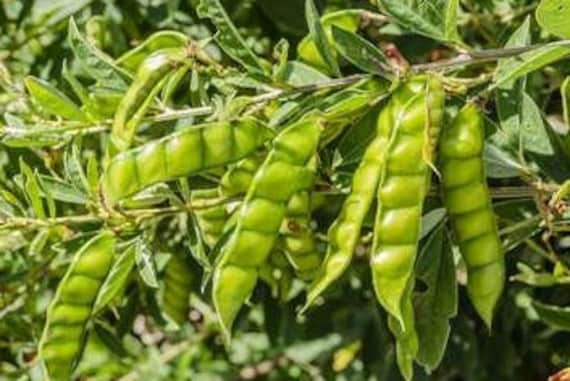The image depicts several green pea pods, likely fava beans, hanging from a horizontally extending branch amid a backdrop of lush green plants. Each pod, gleaming brightly in a rich, shiny green, is elongated and segmented, suggesting the appearance of a centipede but shorter. Typically, each pod contains around five to seven distinct, roundish cavities, marked by indentations and narrowing separations. The peas inside give the pods a segmented look, each ending in a pointy tail. Surrounding these pods are medium-sized leaves, which are greener than the pods themselves, featuring a velvety, rich blue-gray coloring that is characteristic of fava beans.